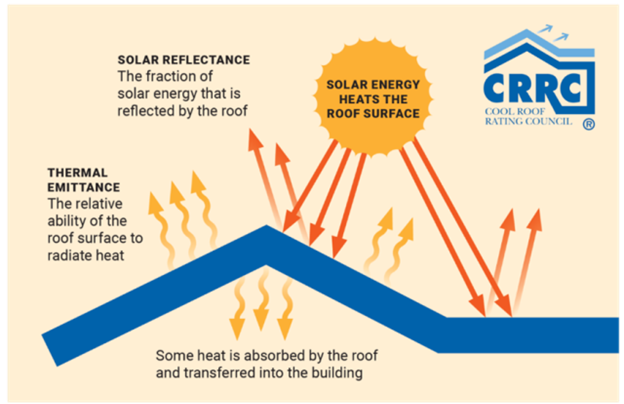The image is a detailed diagram illustrating the interaction between solar energy and a roof surface, designed by the CRRC Cool Roof Rating Council (logo present on the top right). The bottom of the image features a thick blue triangle representing the roof. Above this, a yellow-orange circle symbolizes the sun, labeled with "solar energy hits the roof surface." From the sun, yellow arrows point downwards, indicating the sunlight striking the roof.

Key terms are highlighted: "solar reflectance," describing the fraction of solar energy reflected by the roof, and "thermal emittance," illustrating the roof surface's relative ability to radiate heat, with corresponding yellow arrows pointing upwards. Additionally, there is black text beneath the roof explaining that "some heat is absorbed by the roof and transferred into the building." The overall color scheme includes peach and pinkish hues for the background, yellow for the arrows signifying energy movement, and blue for the roof. The diagram comprehensively conveys the concepts of solar reflectance and thermal emittance in roof surfaces.